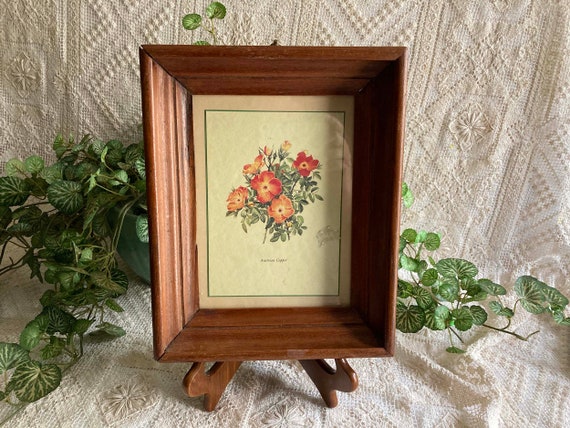This photograph features a vintage botanical drawing of red, orange, and yellow flowers, resembling poppies, with lush green leaves. The artwork is housed in a thick, dark wooden frame about two to three inches wide, positioned on a wooden easel-like stand. The frame sits on a cream textile drop cloth with a geometric pattern, adding a vintage touch. Behind the framed artwork is a faux potted plant with trailing, stylized lily pad-like leaves in green and white, cascading to add depth and greenery. The overall composition blends textures and colors, creating a rich, detailed display. Text under the flowers in the artwork remains illegible, adding an element of mystery to the piece.